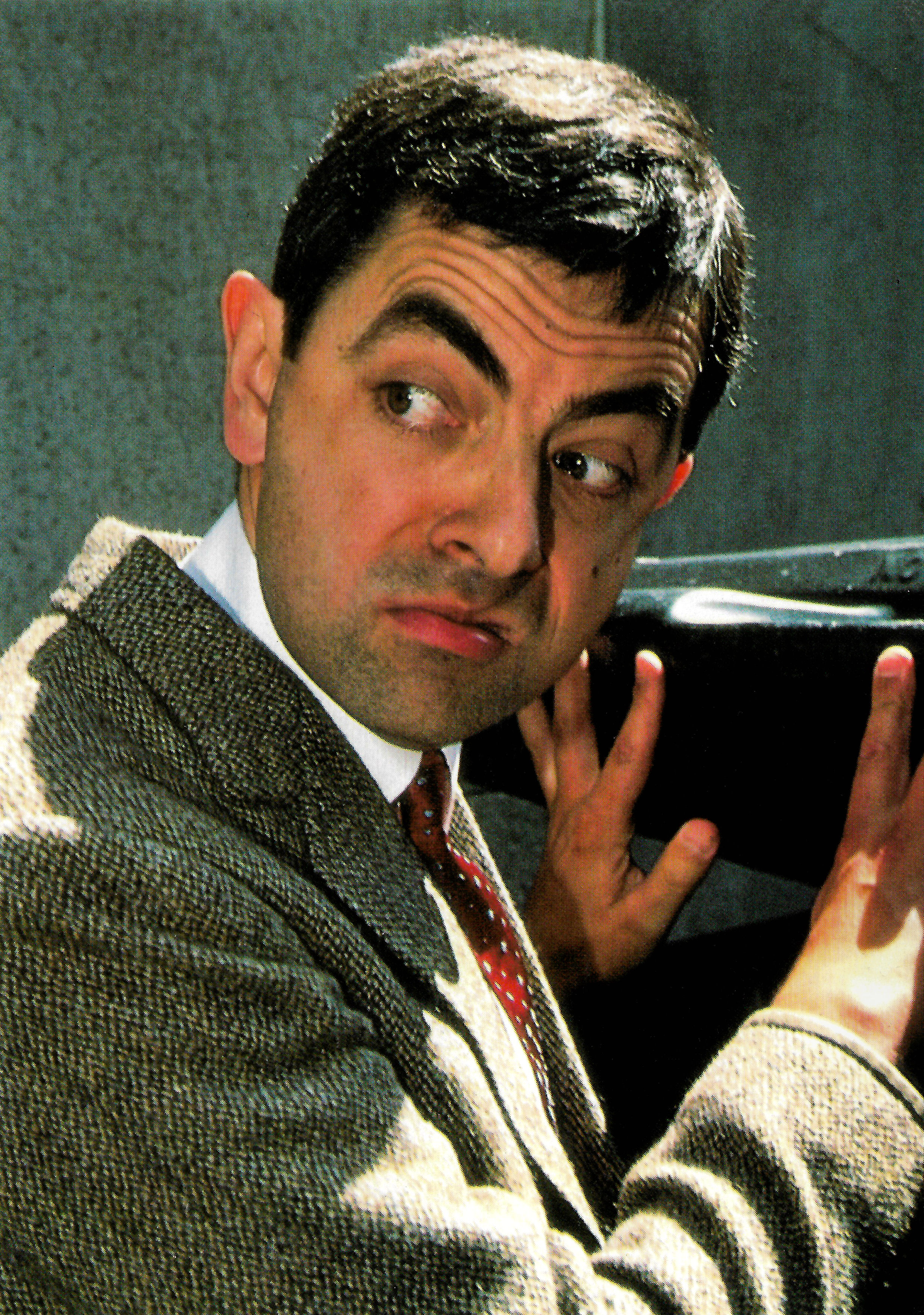The image features the iconic British character Mr. Bean, portrayed by Rowan Atkinson. Mr. Bean is depicted standing in front of what appears to be a dark object, possibly a desk or piano, against a grey, textured backdrop. He is wearing a brown, tweed-like jacket over a white collared shirt and a red tie adorned with white polka dots. His distinctive look includes dark brown hair, prominent ears, and exaggerated facial features, including wide, expressive eyes and a heavily wrinkled forehead. His hands are pressed against the dark object as he turns his head over his left shoulder, wearing a curious, yet worrisome expression with raised eyebrows and a furrowed brow.